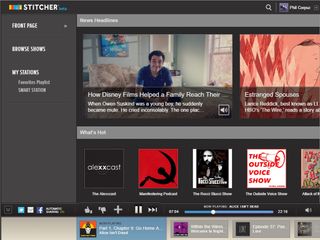This image is a small screenshot from the Stitcher website, an application and platform dedicated to podcast listening. The screenshot features a dark grey background with "Stitcher" written in white text at the top left corner, accompanied by a multicolored logo. Prominently displayed are a few articles with large images. One article includes a picture of a white man with dark hair wearing a blue shirt, sitting in a chair in his living room, alongside a partially visible title that starts with "How Disney Films Helped the Family Reach". Another article titled "Estranged Spouses" features a reddish-tinted image. Below these articles, several small square thumbnails represent various podcast cover arts, though most are illegible; only "The Outside Voice Show" is readable. At the bottom, there is a podcast player interface complete with play, pause, and skip track buttons, providing functionality for listening to podcasts.